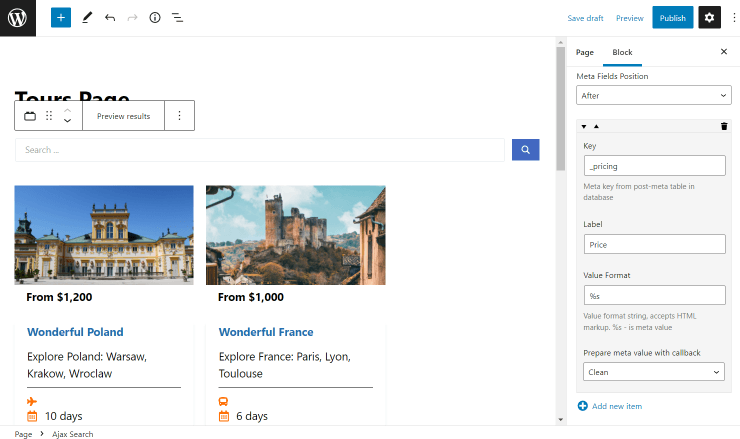The screenshot depicts a WordPress page titled "Tours Page". At the top, there is a calendar, an option to preview the results, and a three-dot menu. Directly beneath is a search bar featuring a blue square with a white magnifying glass icon, indicating its function for searches.

Underneath the search bar, the page showcases two distinct tour packages. 

On the left side, there is an image of a long building reminiscent of a church. Accompanying this image, text indicates a starting price of $1,200 and includes a clickable blue link titled "Wonderful Poland." Below this link, the description reads: "Explore Poland - Warsaw, Krakow, and Wroclaw. A 10-day excursion."

The right side features an image of a castle. The associated text lists a starting price of $1,000 and showcases a clickable blue link titled "Wonderful France." The description underneath states: "Explore France - Paris, Lyon, and Toulouse. This is a six-day adventure."

On the rightmost side of the page, the options "Page" and "Block" are displayed. The "Block" option is currently selected, revealing options related to metafields position, specifically a drop-down menu labeled "After." Additional details include fields labeled "key_pricing," "label_price," "value_percents," and a note about preparing meta value with a callback drop-down menu labeled "Clean."